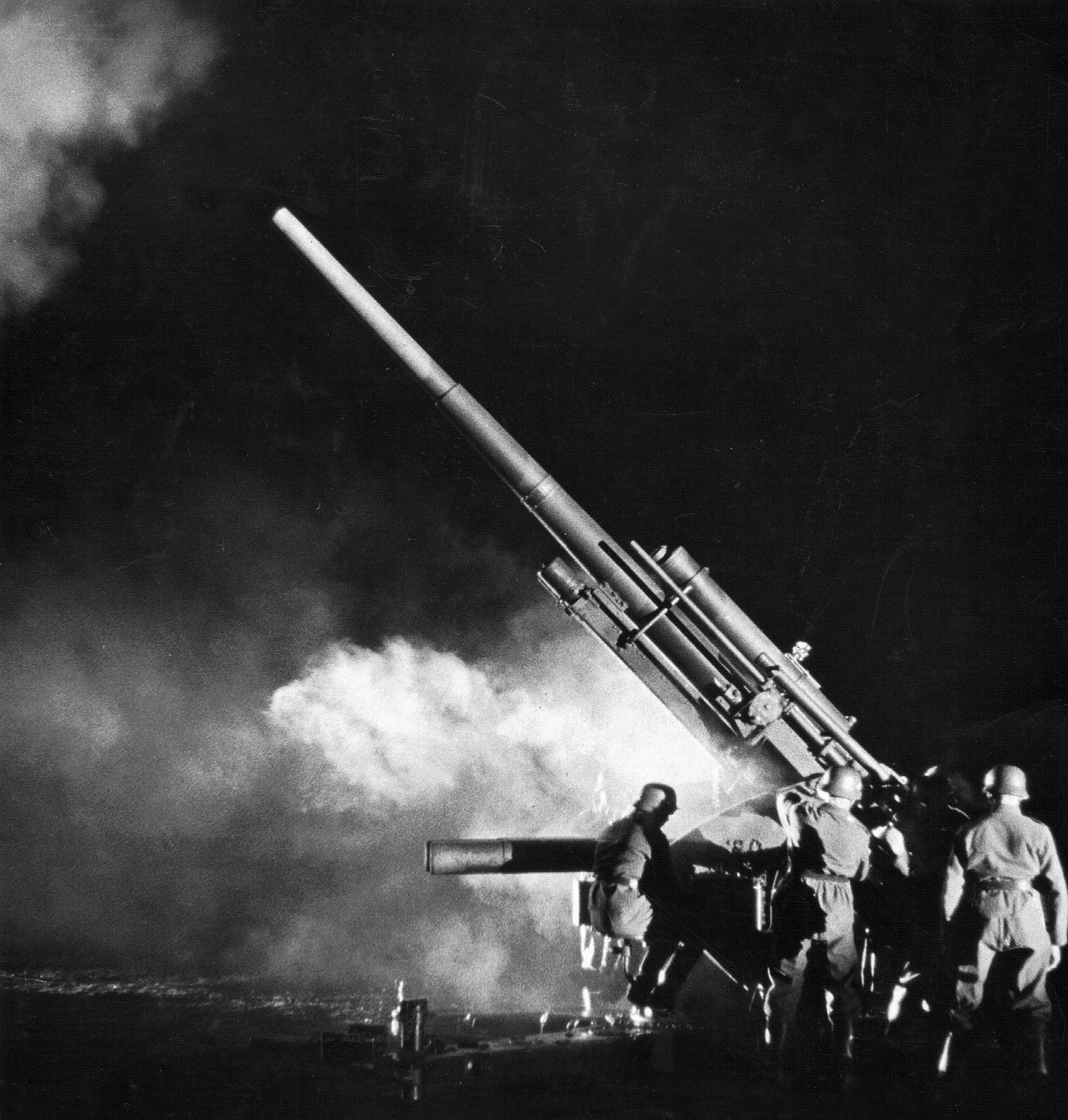In this striking black-and-white photo, likely from World War II, a group of four soldiers, clad in military uniforms and helmets, is seen operating a formidable artillery piece, possibly the feared 88-millimeter German anti-aircraft and anti-tank gun. The scene is enveloped in darkness, suggesting a nighttime setting, with the only source of illumination seemingly emanating from the artillery itself and some distant city lights on the bottom left. The large cannon, with its dark, partially obscured base and smaller attachments near the bottom, extends out at a 45-degree angle towards the top left of the image, its stock aligned with the soldiers. Plumes of white smoke are visible near the bottom middle, adding to the intense atmosphere of an active battlefield. The resolution is low, adding to the photograph's vintage feel, as the soldiers, possibly engaged in the heat of an aerial raid, work with grim determination to keep the massive weapon operational.